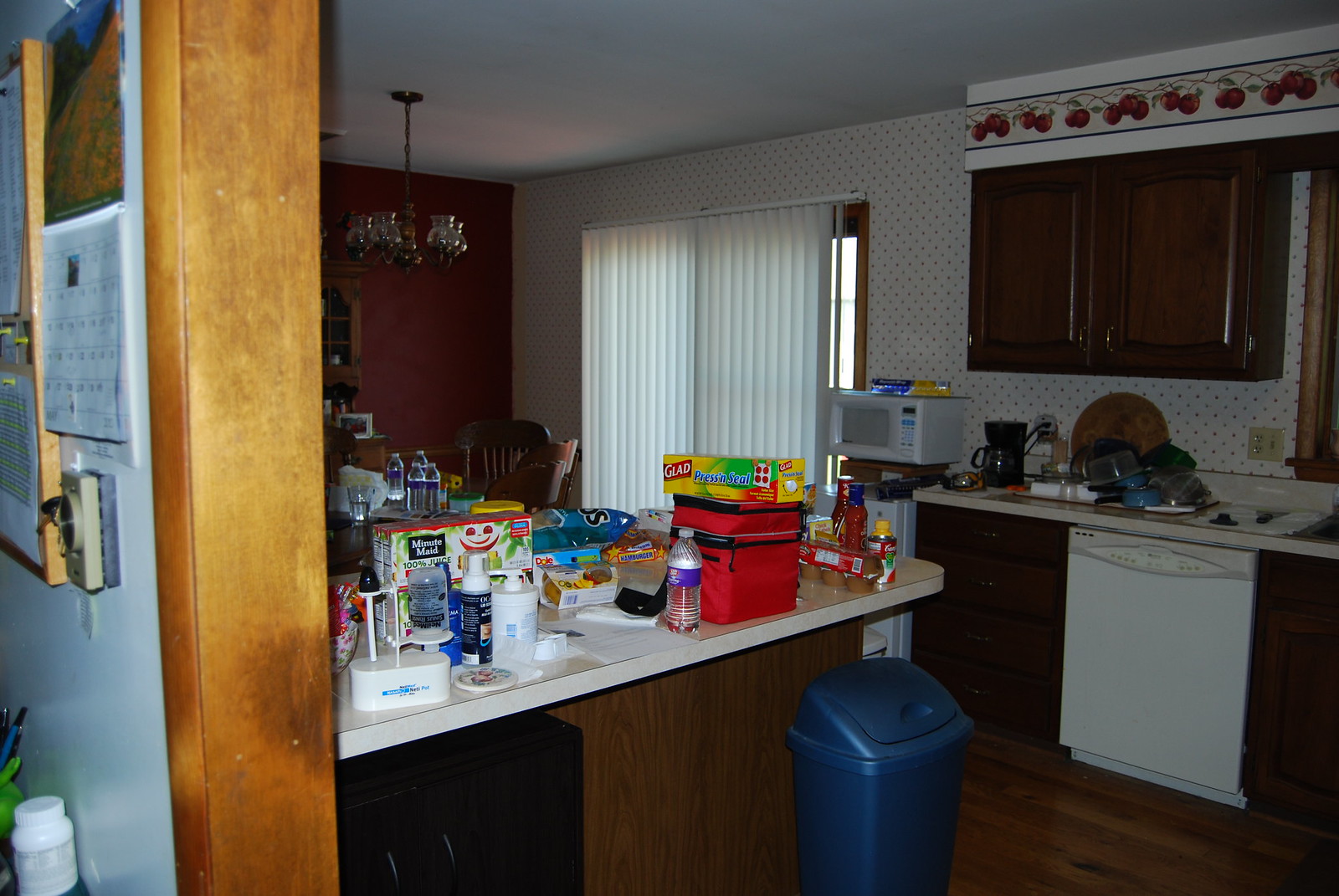The image depicts a cluttered kitchen viewed from an adjacent room in a home, captured in landscape orientation. Natural light filters in through long blinds, which line the windows on the opposite side of the kitchen, casting a soft afternoon glow. A flash appears to accentuate the scene, revealing the countertops strewn with various food items, packages, and water bottles, contributing to an overall disorganized appearance. Beneath the countertops, a blue trash bin with a matching lid is visible. The wooden cabinets frame the room, adding a warm, rustic touch. Towards the far end of the kitchen, one wall stands out with its brick red color, adorned by a hanging chandelier. On the other side, a stark white dishwasher is situated among black cabinets, adding a stark contrast. The countertop above the dishwasher is cluttered, mirroring the mess seen throughout the kitchen.